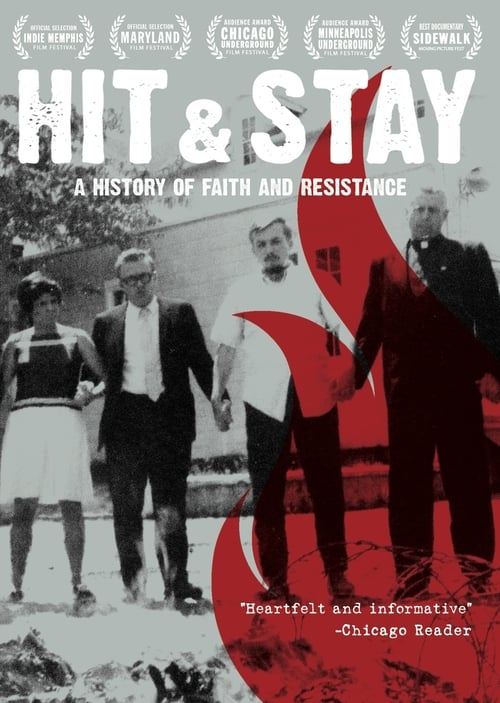The image is a detailed movie poster resembling a Blu-ray or DVD cover, featuring a bold black-and-white photograph at its center. The black-and-white image showcases four people standing hand-in-hand in front of a white house on a lawn. They include a woman on the left, wearing a sleeveless black top with white stripes and a knee-length white skirt; next to her, a man in a dark suit, white shirt, and a light-colored tie with glasses; beside him, a man in an untucked white short-sleeved shirt and black pants; and on the far right, a man in a dark suit with a clerical collar, appearing to be a priest.

At the very top of the poster, there are several symbols indicating awards the movie has garnered, specifically from festivals such as the Memphis Maryland Film Fest, Chicago Underground Film Fest, Minneapolis Underground Film Fest, and Sidewalk Film Fest. These accolades are displayed in white text framed by olive branches.

Below the awards, in large white bubble letters, the title "Hit & Stay" is prominently displayed, with the subtitle "A History of Faith and Resistance" in smaller white font beneath it. 

On the right side of the poster, a red flame graphic is superimposed, adding a striking visual element. In the lower right corner, there is a quote in white text reading, “Heartfelt and informative,” attributed to the Chicago Reader, enhancing the credibility and emotional appeal of the film.